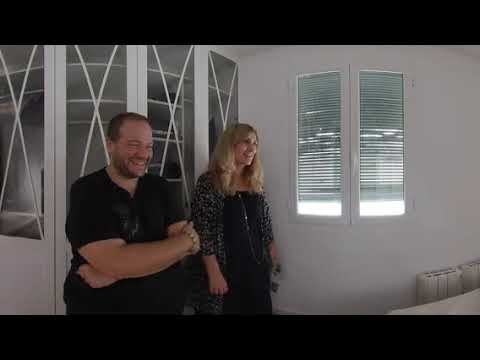In this image, a man and a woman stand side by side, both smiling and laughing, creating a cheerful atmosphere. The man, positioned on the left, sports a black T-shirt adorned with sunglasses hanging from the collar, a beaded bracelet on his wrist, and has brown short hair with light facial hair. He stands with his arms crossed and appears slightly heavyset. To his right is a woman with long blonde hair, wearing a black dress with a cheetah-patterned shawl. They both radiate middle-aged warmth and share a familial resemblance, possibly siblings.

The scene is set indoors, in a room with pristine white walls. Behind them is a tall, white cabinet with cross-hatched glass doors, adding a textured detail to the otherwise plain background. The room’s sole window is mostly covered by blinds, allowing only a sliver of sunlight to filter through. To the right, slightly out of focus, there is either a white table or a heater, contributing to the all-white decor of the surroundings. This monochromatic setting sharply contrasts with the dark clothing worn by the two individuals, focusing attention on their bright expressions.